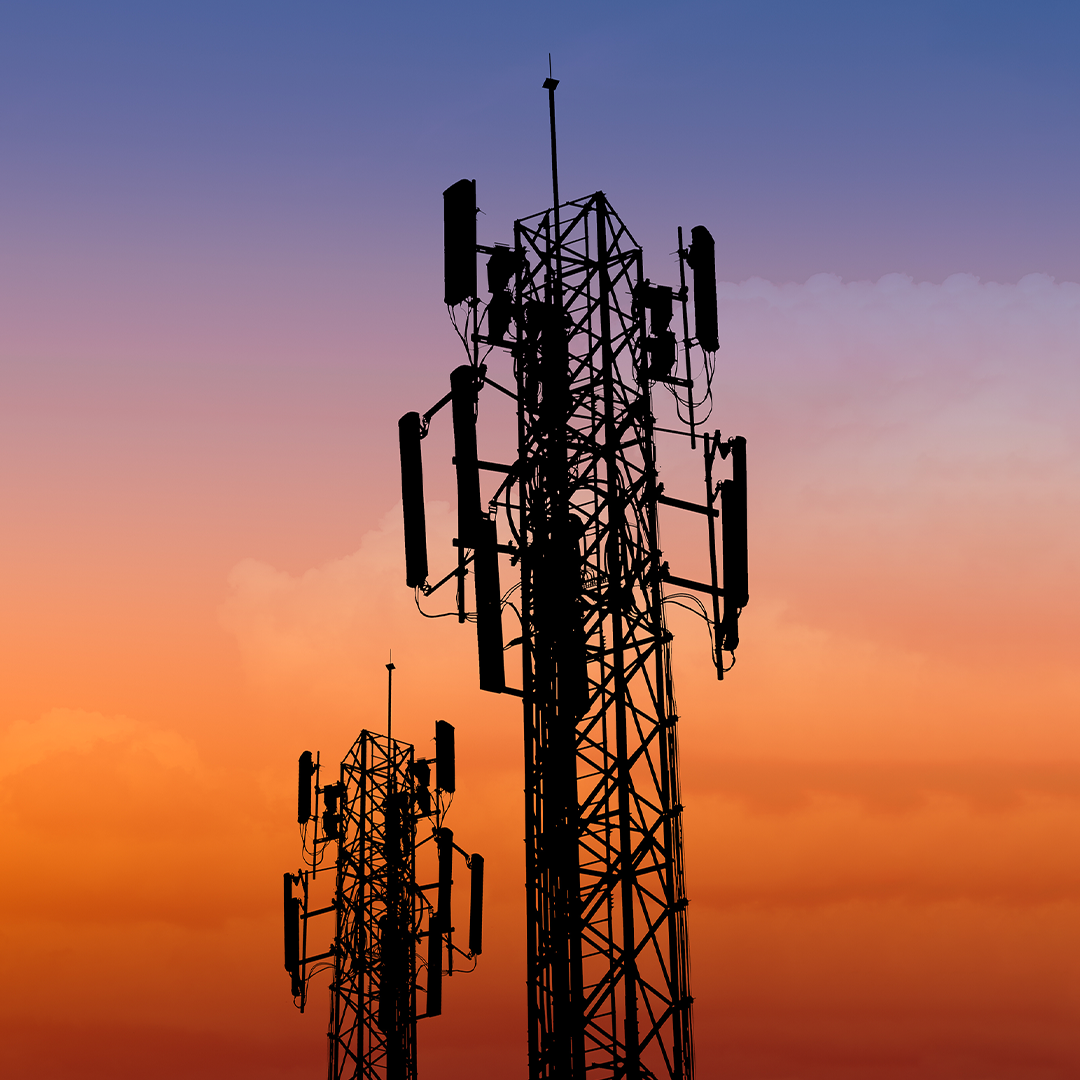This photograph, taken outdoors during either early morning or late evening, showcases a stunning sunset that transitions from a rusty red at the horizon through various shades of orange and peach to a violet and dark periwinkle blue sky. Central to the composition is the silhouette of two identical 5G cell phone towers. The closer tower stands in sharp relief, while the second, situated slightly to the left and further back, appears smaller due to its distance. Both towers feature a long, boxy metal structure with a central ladder, crowned by antennas and festooned with long, rectangular attachments for signal reception and boosting, resembling small speakers or grenades hanging from their tops. The towers are constructed with a stable, crisscross pattern of metal supports, adding to their imposing, industrial presence against the colorful backdrop.